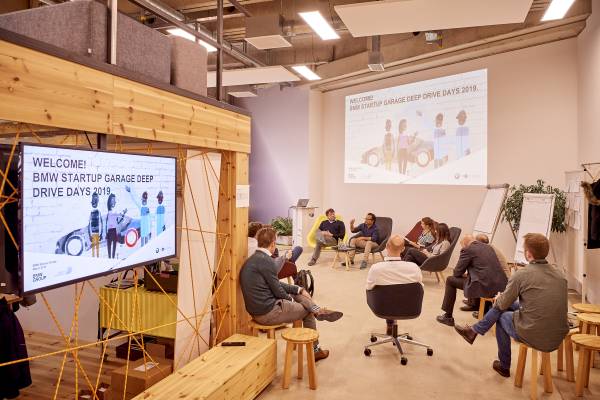The image depicts a large office or warehouse setting configured for a meeting or class, likely related to BMW's Startup Garage Deep Drive Days 2019. The room features high ceilings with overhead fluorescent lighting, light tan walls, and a floor covered in matching tan carpet or tile. On the left side is a natural-looking wooden structure resembling a bench, topped by horizontal bars suggestive of an unfinished or industrial space. A prominent poster hangs here, reading, "Welcome BMW Startup Garage Deep Drive Days 2019," accompanied by a cartoon graphic of a car and four people.

In the middle and right side of the room, participants are seated in a mix of seating arrangements: lightweight wooden stools and a few dark brown padded chairs. The attendees wear casual business attire, such as slacks or jeans paired with nice shirts. The central focus of their attention is a rectangular projected image on the upper right wall that echoes the content of the poster: "Welcome BMW Startup Garage Deep Drive Days 2019," with a similar cartoon graphic of a car and figures. Additional details include large paper pads on stands, suggesting a workshop or collaborative meeting atmosphere.